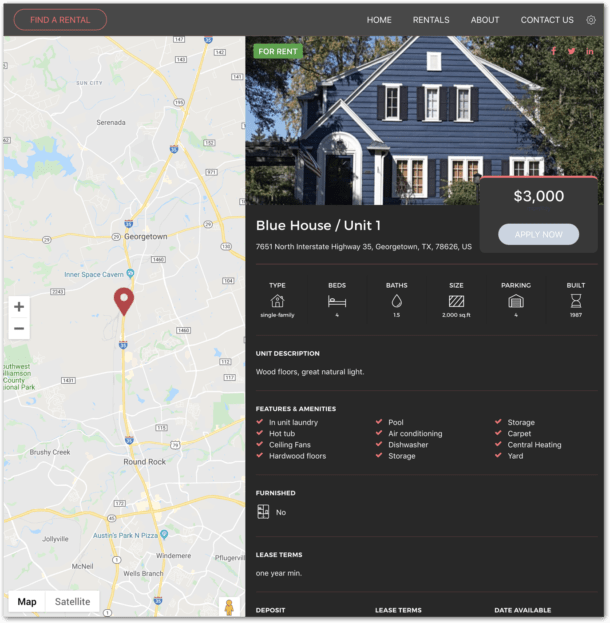In this image, we observe a screenshot featuring a comprehensive layout of a rental listing. At the upper left corner, against a dark gray banner, bold red text reads "Find a Rental." To the right of this banner, white text displays navigation options, including "Home," "Rentals," "About," and "Contact Us," accompanied by a settings icon.

The left side of the image showcases a detailed map. The map has a light tan backdrop with white roads, yellow highways, and interstates. Key locations are marked: "Inner Space Cavern" in blue text at the center, and "Georgetown" in black text just below. Other labeled areas include "Round Rock," "Wells Branch," "Windermere," "Jollyville," and "McNeil."

On the right side of the image, there is a photo of a charming blue two-story house surrounded by lush trees. The text near the house reads: "Blue House Unit 1 - $3,000. Apply Now." Below this are the address details: "7651 North Interstate Highway 35, Georgetown, Texas, 78626, U.S."